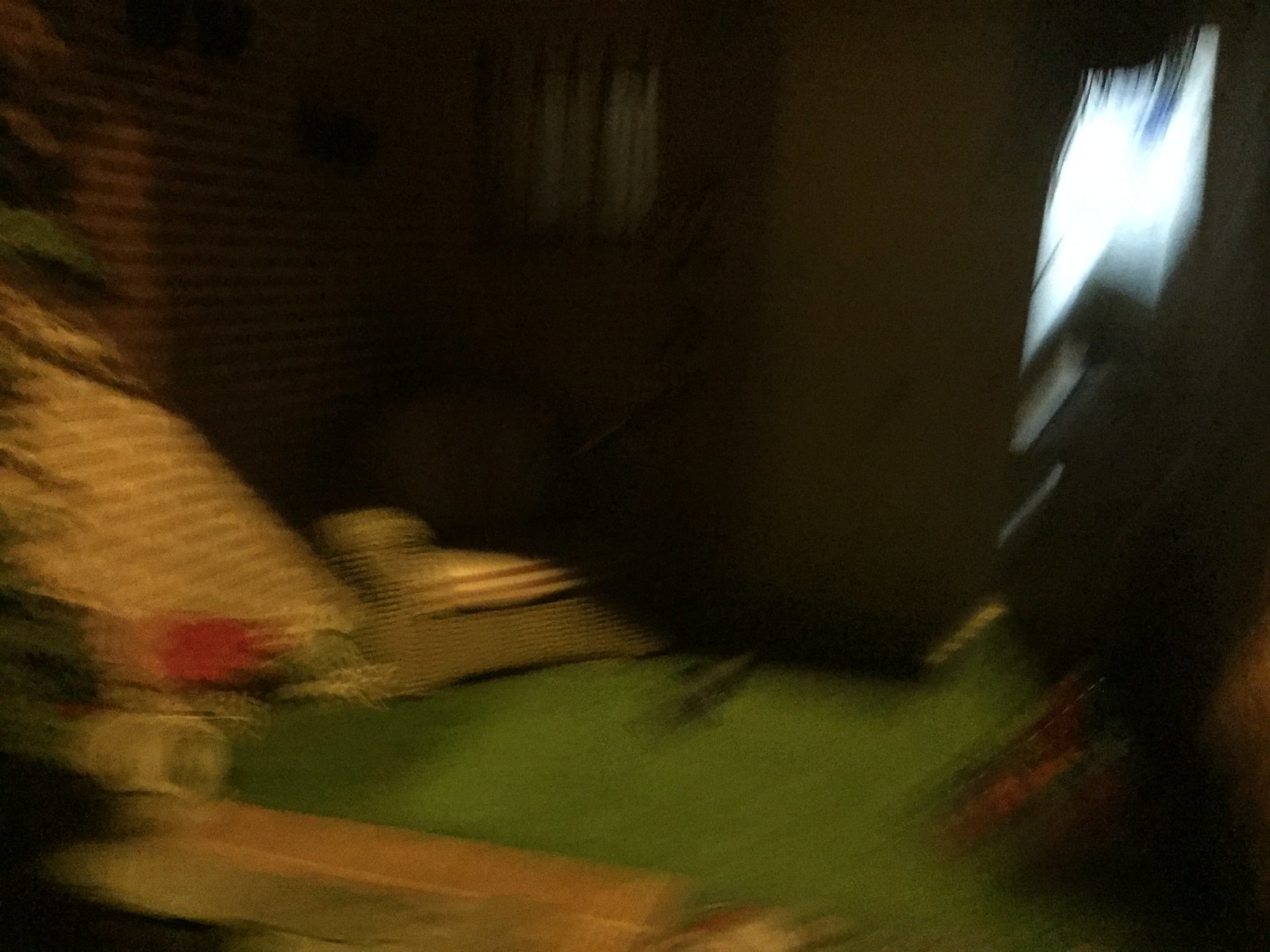This image depicts a slightly blurry scene of what appears to be a bedroom. Central to the scene is a bed, either resting directly on the floor or on a very low frame, draped with a green blanket. The overall image lacks sharpness, contributing to the indistinct outlines of various objects. 

In the background to the right, there's an open doorway emitting light, which illuminates part of the white wall to its left. Further to the left, near the back corner of the room, a small square of light suggests the presence of a window. Positioned beneath this possible window is a round, fluffy object that resembles a bean bag, adding a cozy element to the room's decor. 

On the left side of the photograph, a white piece of furniture with stripes is partially visible, which could be interpreted as either a chair or a couch, adding to the room's furnishings. The overall ambiance suggests a casual, lived-in space with a mix of functional and comfortable elements.